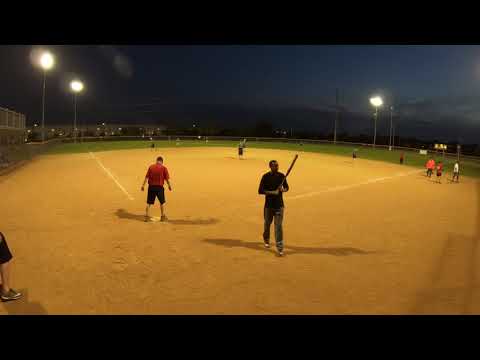This photograph captures a nighttime baseball game from a vantage point behind and slightly to the left of the catcher. The field is illuminated by bright stadium lights, casting multiple shadows from each player across the golden-yellow dirt of the infield and the lush green grass of the outfield. The deep navy-blue sky suggests it is either late evening or just transitioning to night. The players seem to be in casual attire rather than official jerseys, with one batter in a red t-shirt and black shorts at home plate and an umpire in a red shirt with black pants cleaning the base. Another player, dressed in a black t-shirt and grey jeans, is seen walking back from the plate holding a bat. Additional players can be seen scattered around the field and on the sidelines, underscoring the informal atmosphere of the game.